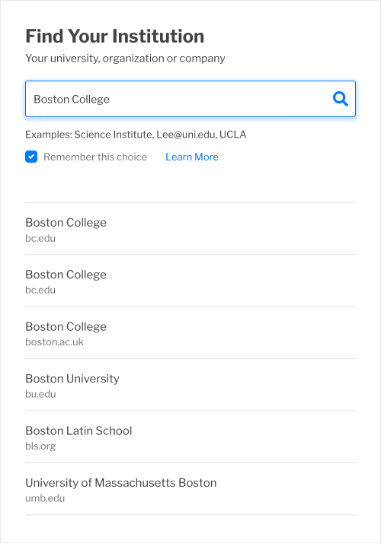The image in portrait format is a color screenshot of a mobile website or app designed for users to locate their institution. At the top, a bold header reads, "Find your institution, your university, organization, or company." Below this, a search bar is available for user input. 

In the image, the user has typed "Boston College" into the search bar and checked the option "Remember this choice." The search results displayed beneath the input field include a variety of institutions related to the query:
- Boston College (bostoncollegebc.edu)
- Boston College (boston.ac.uk)
- Boston University (bu.edu)
- Boston Latin School (bls.org)
- University of Massachusetts Boston (umb.edu)

Before the user entered their query, examples like "Science Institute" (lee.uni.edu) and "UCLA" were provided to illustrate the type of searches users can perform.

The app or website appears to be a tool for retrieving the domain names associated with different educational and organizational institutions, potentially for purposes such as finding official email addresses or gathering more information about each entity.